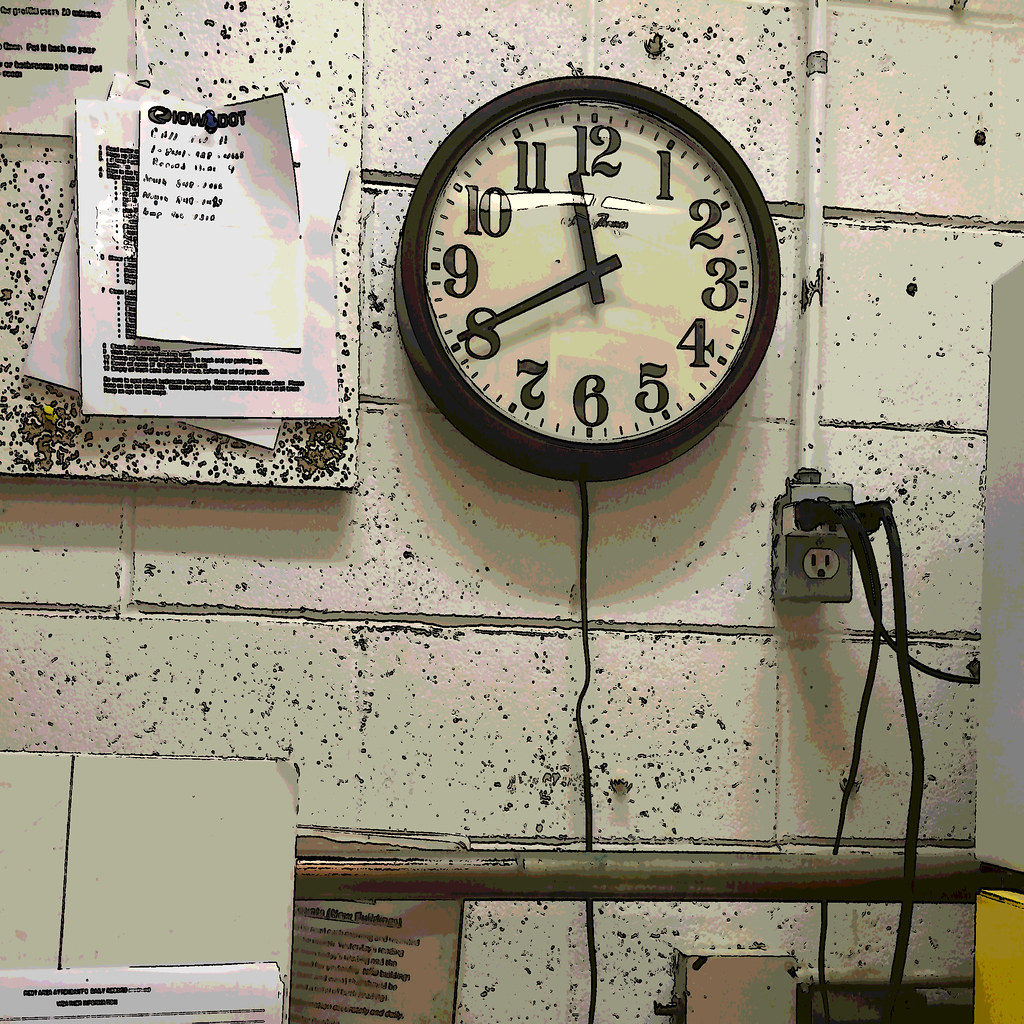A highly detailed and lifelike animation depicts a square-shaped scene of a white concrete wall. Prominently featured in the center of the wall is a sleek black clock with a white face, displaying the time as 11:40. To the left side of the wall, a bulletin board is adorned with several flyers, adding a touch of everyday realism. On the right side, an electrical outlet has two cords neatly plugged in, providing a sense of functionality to the scene. Further to the right, there's a small, indeterminate silver object mounted against the wall. Along the lower edge of the image, a polished silver bar extends horizontally from left to right, grounding the composition and contributing to the overall realistic quality of the animation.